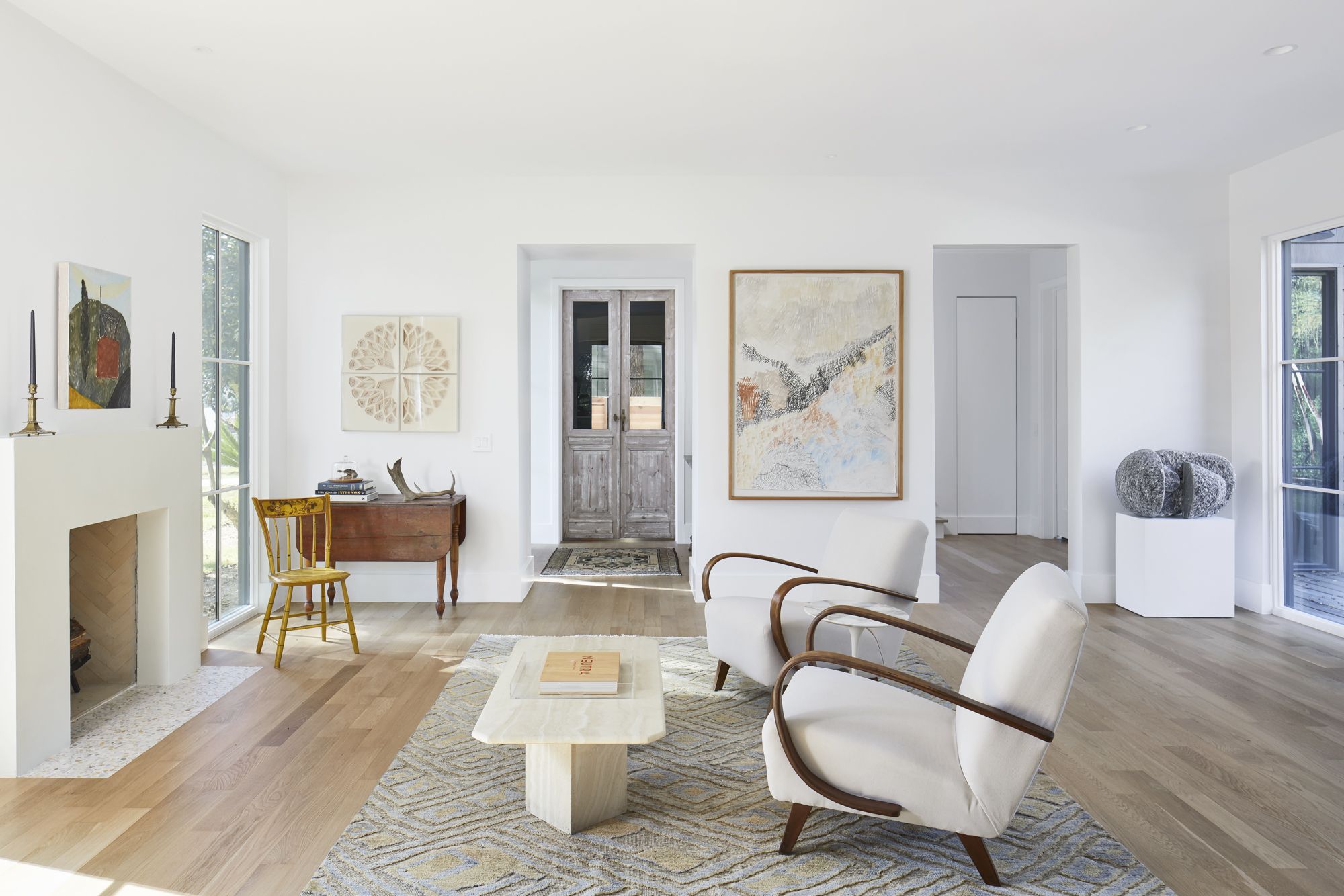This image features a clean and minimalistic living room with light brown hardwood floors. Central to the room is a textured gray rug upon which rest two white chairs with wooden legs and handles, positioned around a small white wooden coffee table with a book on it. To the left of this setup is a striking white marble fireplace adorned with two candlesticks on the mantle and a painting above. The room is decorated with multiple pieces of art on the walls, enhancing the aesthetic. Notably absent is any electronic device, adding to the refreshing simplicity of the space. In the background, two open doorways lead to other parts of the house, and two wooden doors are visible, potentially leading outside. A darker brown wooden desk resides against the back wall with another piece of art above it. Additionally, a yellow wooden chair is positioned by a large window, adding a pop of color to the serene setting. Various rugs and a mix of modern and antique furniture complete the inviting look of the room.